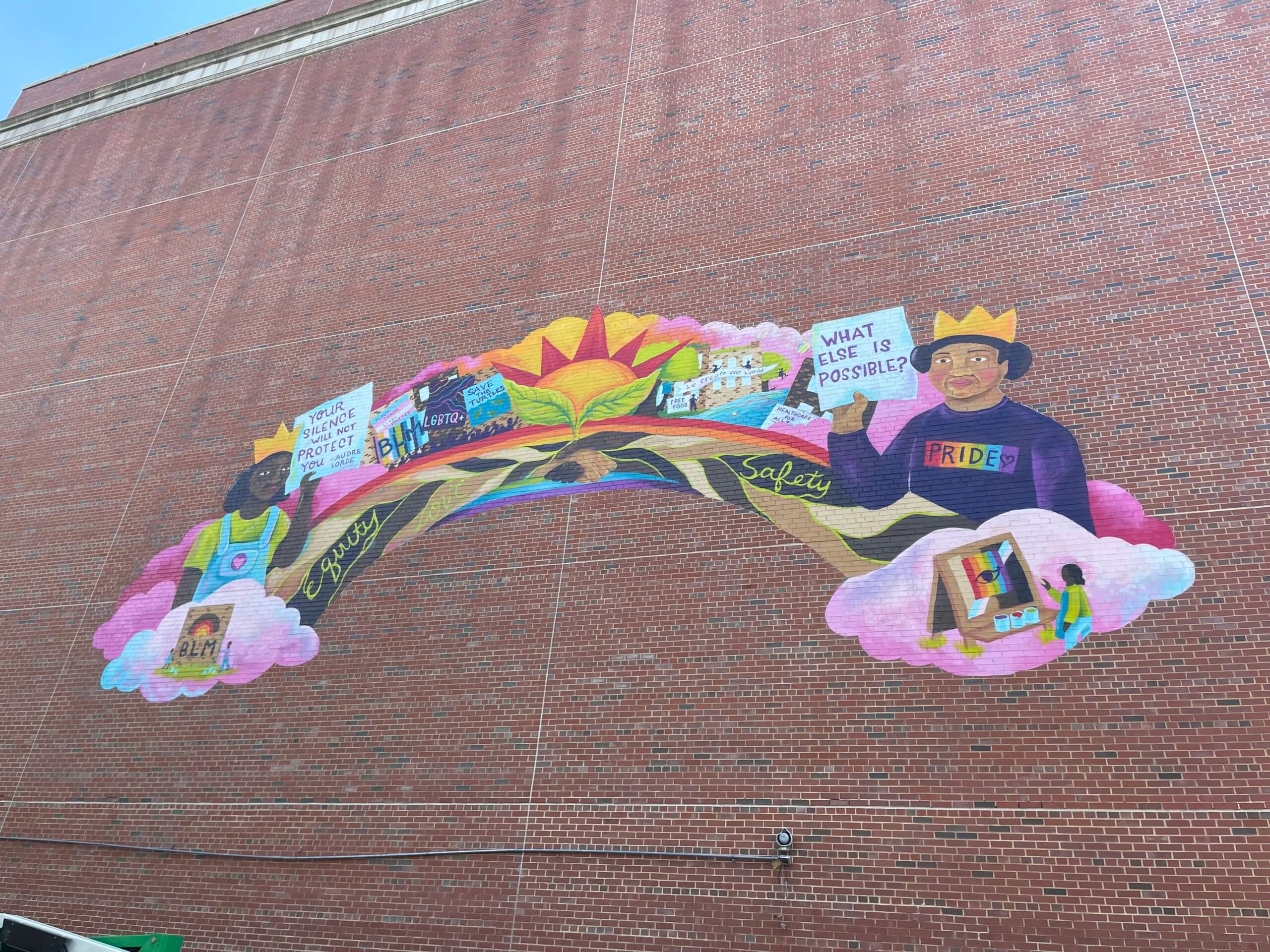The image showcases a large red and black brick building with a mural on its side. The mural features a prominent rainbow arch connecting two figures—a black woman on the left and a man on the right, each wearing yellow crowns. The woman, dressed in a purple shirt with the word "Pride" emblazoned across it in rainbow letters, is holding a sign that reads, "What else is possible." The woman on the left wears a purple shirt and also sports a crown, holding a sign that says, "Your silence will not protect you." In the center of the rainbow is a sun with red rays and two leaves cradling it. Above the sun, there's a snippet of blue sky peeking through the top left corner of the image, indicating it's daytime. Additional words such as "Equity" and "Safety" are visible around the mural. There are no windows on this wall, only small white dividing lines marking different sections of bricks, and there's an electrical wire running horizontally near the bottom of the image.